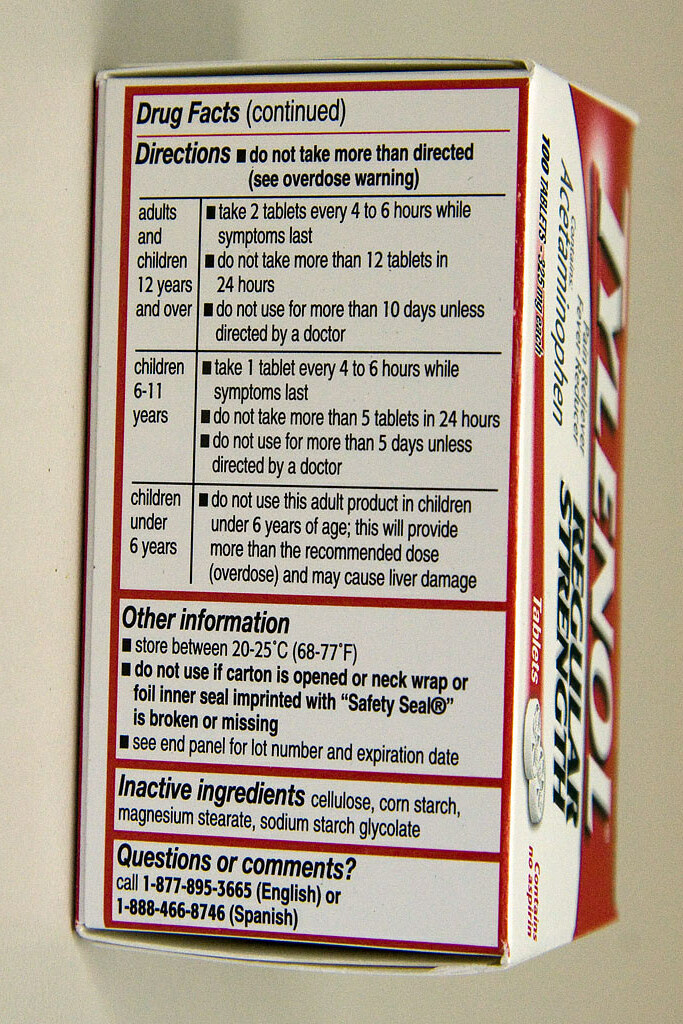The image features the side of a medication box labeled "Tylenol, Regular Strength" with the active ingredient clearly stated as Acetaminophen. Information on the side of the box presents extensive drug facts, including detailed usage directions and dosage guidelines for adults and children aged 6 to 11 years, as well as precautions for children under 6 years. Additional details such as optimal storage temperature, instructions on what to do if the medication seal is broken, and an expiration advisory are visible. Further, the box lists inactive ingredients like cellulose, cornstarch, magnesium stearate, and sodium starch glycolate. There are also sections for consumer questions or comments, providing contact numbers for both English and Spanish speakers. The text on the side of the box is outlined with a red border, and the "Tylenol" brand name is set against a red background.